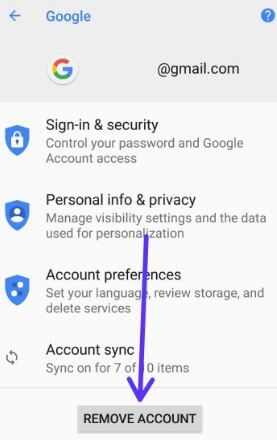The image depicts a Google settings menu. At the top left corner, you can see the Google logo. In the top right corner, there is a blue circle featuring a white question mark, likely a help or support button. The email address associated with the account has been fully removed, presumably for security purposes.

Below this, the menu is divided into several categories:
1. Sign-in & Security
2. Personal Info & Privacy
3. Account Preferences
4. Account Sync

A prominent purple arrow starts just below the "Personal Info & Privacy" section, pointing towards the bottom of the screen. It indicates an option labeled "Remove Account," which is displayed with black text inside a gray box. The caption suggests that the user might be intending to remove their Google account from their device using this setting.